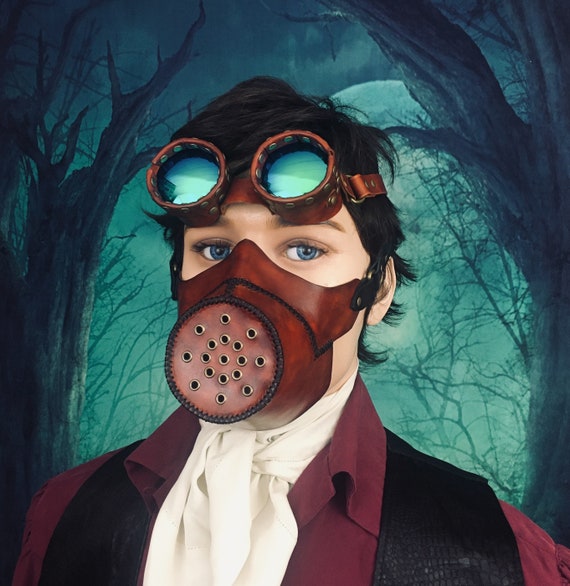In this incredibly detailed and surreal image, a man stands as the central focus, clad in steampunk attire that vividly contrasts with his eerie surroundings. He wears a distinctive gas mask crafted from leathery brown burgundy material, featuring numerous metallic holes for ventilation. This mask covers his pale face and is topped with reflective glass goggles resting just above his brow. The man's hair is a mix of medium-length black with hints of blue, adding to his mysterious appearance.

He is dressed in a layered outfit consisting of a white dress shirt underneath a vibrant red coat, and a black scaly vest draped over his shoulders. The intricate detailing of his attire is complemented by the background, which has an almost painted quality to it. 

The background presents a spooky, dark night scene with a luminescent moon casting a ghostly light over a forest of barren trees, their branches arching in various directions to create an unsettling atmosphere. The contrast between the crisp, almost photographic quality of the man and the darker, more surreal background creates a striking visual impact. This juxtaposition enhances the overall sense of mystery and foreboding that the image evokes.